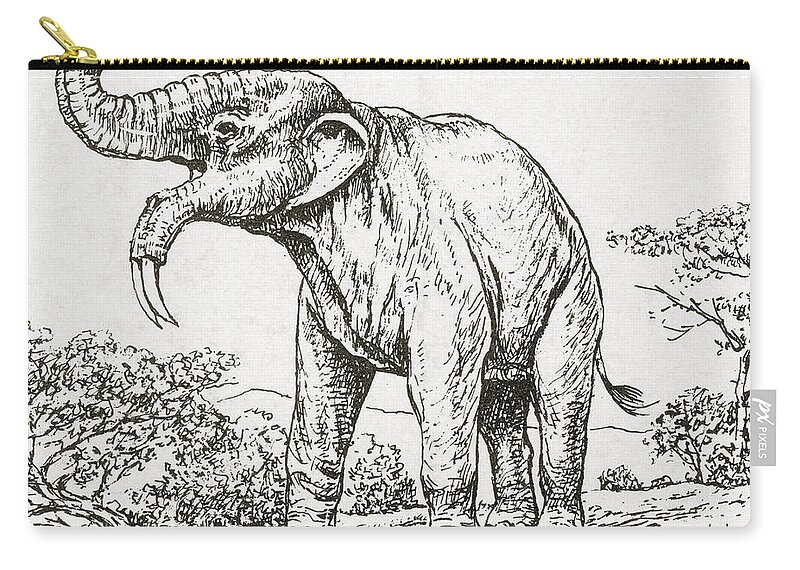The image showcases a small bag, potentially used as a pencil case, makeup bag, or storage pouch, set against a pure white background. The bag itself appears to be made of canvas or a similar cloth material and features a top zipper with black trim and brass or gold zipper teeth. The central design on the bag is a black ink drawing with a pen-drawn style, depicting a detailed elephant with its trunk raised. The elephant, resembling an African elephant with smaller ears and two tusks curving downward from its open mouth, is surrounded by elements of a natural landscape including hills, trees, and bushes. The animal is walking towards the left with its tail visible, possibly swatting at flies. In the bottom right corner of the bag, there is a gray text box with the words "PX Pixels" written in white font, likely denoting the brand.